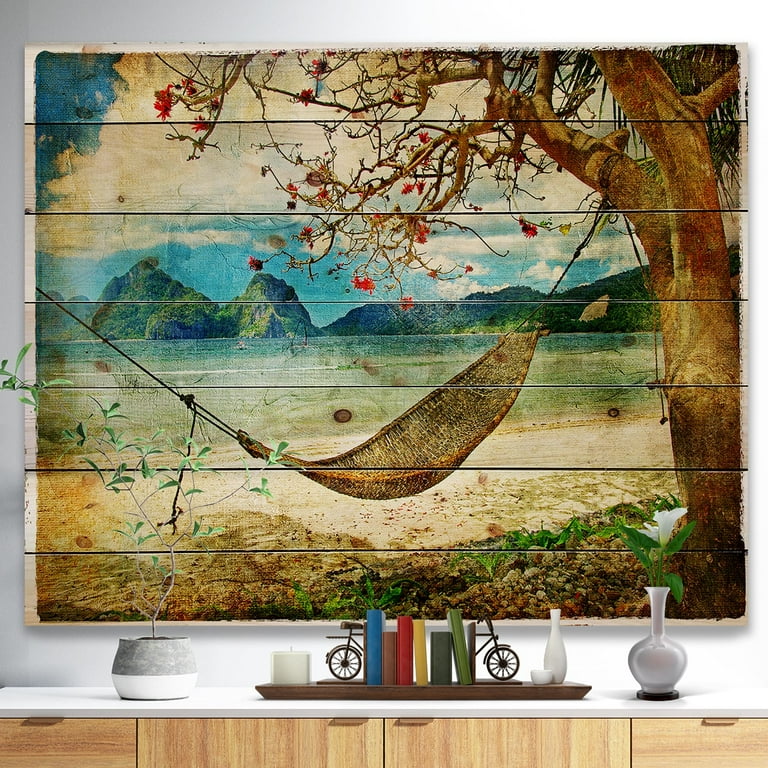The image features an intricately detailed interior living room with a distinct digital art piece as its focal point. The majority of the wall is adorned with a weathered, antique-like painting set on slats of wood, depicting a serene beach scene. Central to the artwork is a brown hammock tied to a tree with red blossoms, shedding its leaves. The scene transitions from sandy shores to calm waters that darken towards the horizon, and in the background, large, rocky hills rise under a beautiful blue sky with fluffy white clouds.

Underneath this captivating painting is a wooden sideboard with brass handles. It is meticulously arranged with a variety of decor: a few vases, a lit candle, a set of books held by bicycle-shaped bookends, and a small plant in a gray and white vase on the left side. Also present is a wooden tray enhancing the curated, stylish appeal of the room. The composition creates a calm and inviting atmosphere, blending the rustic charm of the artwork with the elegant decor of the furniture.